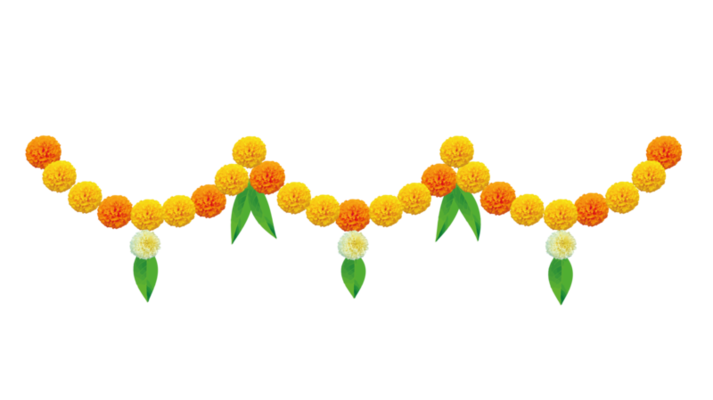This is an image of a decorative floral garland, horizontally laid out against a solid white background. The garland forms three scalloped arches that dip down and back up from the upper left-hand corner, through the middle, to the right. Composed of alternating orange, yellow, and lighter orange pom-pom-like flowers, the pattern repeats consistently with two yellow flowers between each orange one. At the bottom center of each arch, there is a white flower accompanied by a green leaf. Furthermore, where each arch connects, there are pairs of green leaves. The overall arrangement gives an impression of a vibrant party or spring decoration, though the supporting chain or thread is not visible in the image.